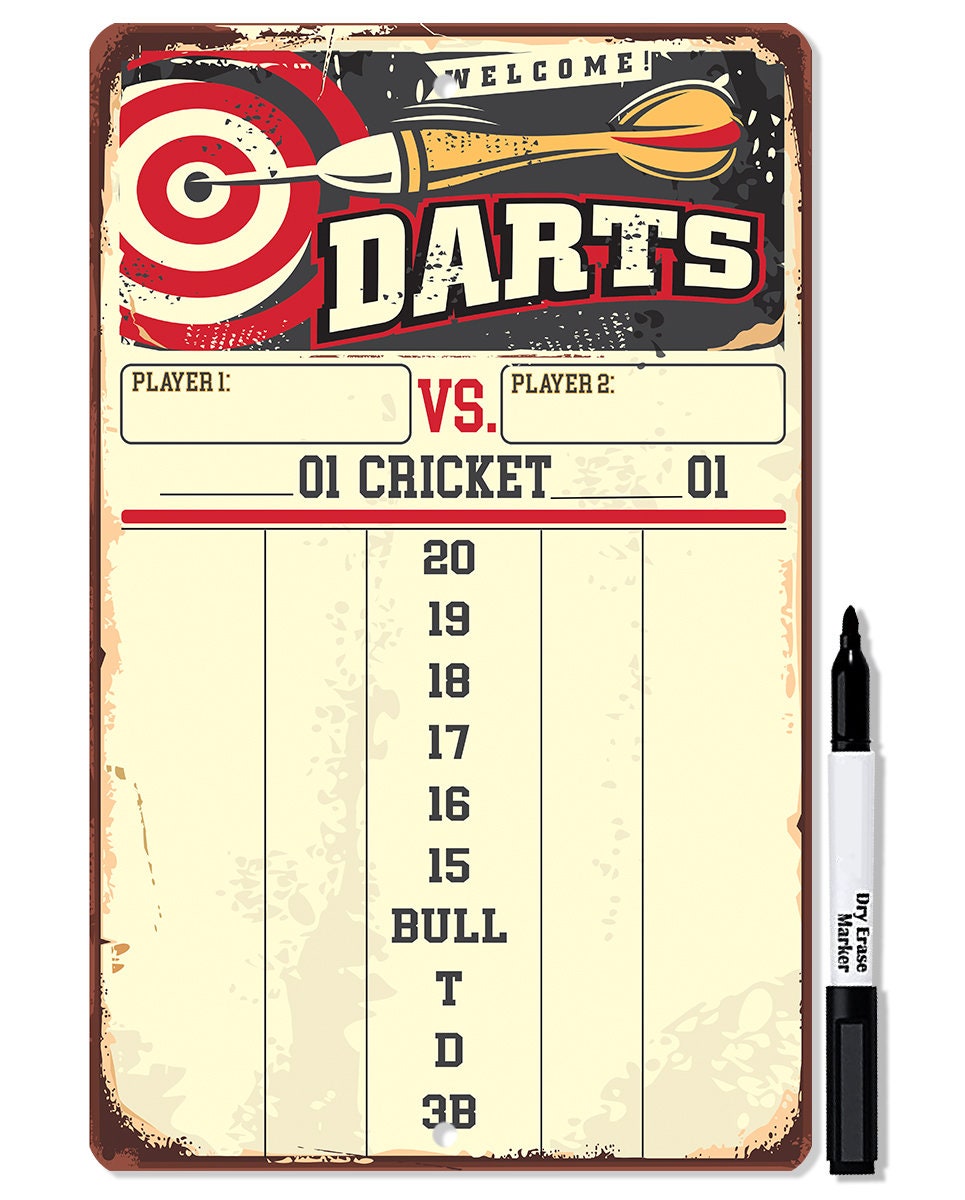A detailed photograph in portrait mode features a retro 1950s-60s style dart game scorecard. Dominating the top section is the word "Welcome" followed by a striking image of an orange dart piercing the bullseye of a red, white, and black target. Below this, "DARTS" is prominently displayed in white font with red and black outlines. The scorecard includes two outlined rectangles labeled "Player One" and "Player Two," separated by a red “VS.” Directly beneath, it reads "Zero One Cricket - Zero One," and further down is a five-column table listing the standard dart scoring numbers: 20, 19, 18, 17, 16, 15, Bull, T, D, 3, B. The card shows signs of wear with rust around the edges. To the right, an uncapped dry erase marker rests on its cap; the marker's body is white with black tips.